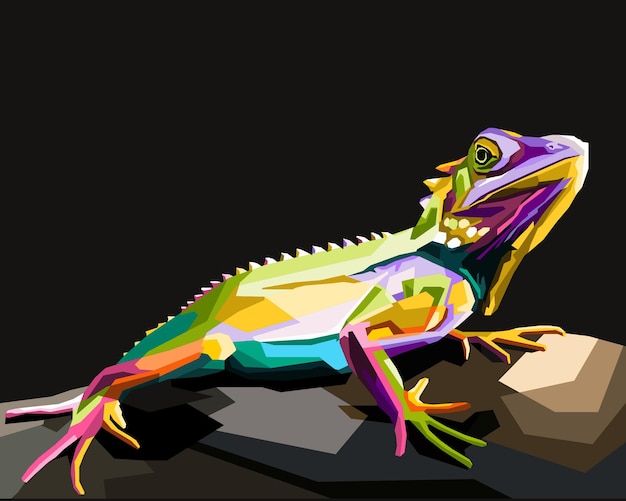This digital artwork features a vividly multicolored iguana sprawled across an arrangement of abstract, geometric rock shapes, all set against a flat black background. The iguana predominantly occupies the image’s width, with its body oriented to the right. It has its head slightly tilted, allowing for a partial frontal view of its snout, yet only one side of its face is visible. The iguana is a kaleidoscope of colors, including yellow, purple, and green. Its back is adorned with small spikes, and its tail showcases a striking pink hue. Its front legs are green with toes that are color-coded: two green, one pink, and one orange. The entire iguana is composed of sharply delineated, angular shapes, each color distinctly separated without blending into the others.

The iguana rests upon rocks designed to look both abstract and geometric, composed of shapes like trapezoids, hexagons, and octagons, all with uneven edges and vector-like precision. These rocks feature a range of colors, including khaki, brown, dark brown, and gray, paired with harsh shadows in darker shades of the same hues. The iguana’s eyes are completely black, while the snout contains a touch of purple, and the underside of its mouth is marked by a bold yellow, complete with a visible nostril detail.